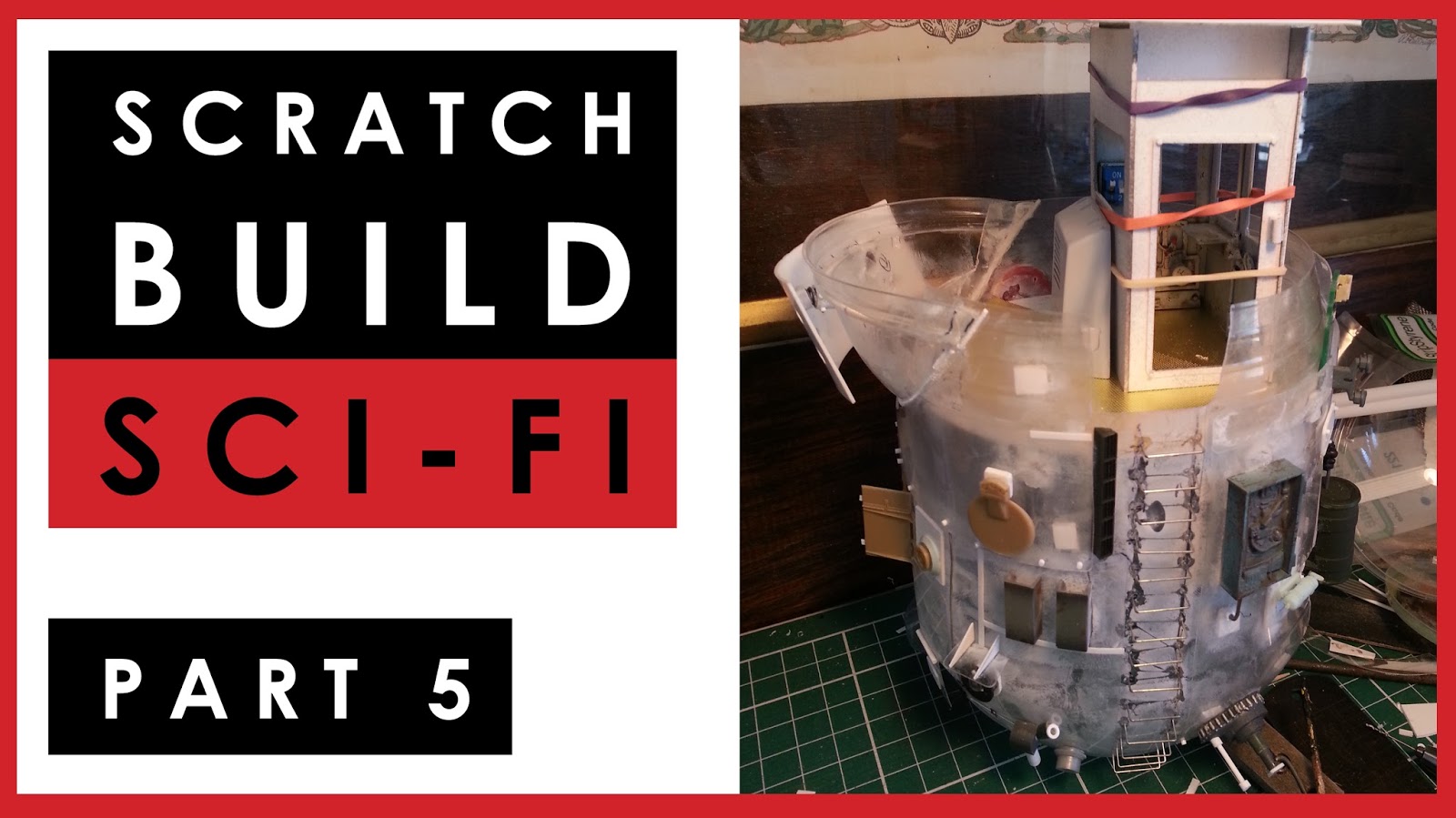This image, titled "Scratch Build Sci-Fi Part 5," features a bifurcated layout with text on the left and a picture on the right. The left side has a black background with bold white text reading "Scratch Build" and red text beneath it stating "Sci-Fi." Below, in smaller white text on a black background, it reads "Part 5." The right side displays a detailed photograph of a handmade gadget. This contraption has a cylindrical base with a structure that resembles a wire ladder on its front. Atop the base rests a rectangular transparent component, possibly fashioned from paper or cardboard, resembling a miniature clear phone booth. The device is secured with three rubber bands in beige, red, and purple colors. To the left of the gadget is a plastic piece designed to catch or pour liquids, characterized by its rounded shape. The entire assembly is situated on a green and white measured grid, reminiscent of a cutting board or a lab surface, contributing to the scientific or instructional theme suggested by the image.